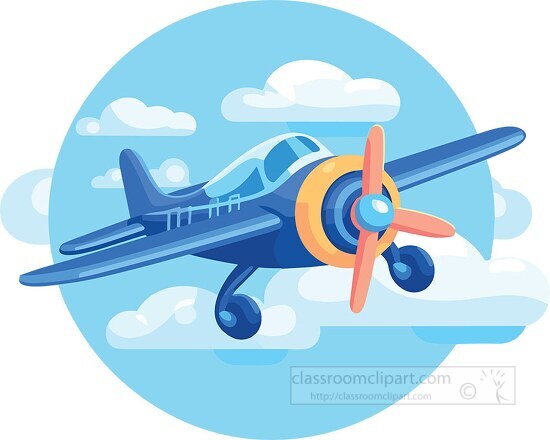This detailed illustration depicts a dark blue cartoonish airplane with a much lighter, almost white cockpit. The airplane has a distinctive propeller comprising three blades positioned in an unusual configuration, with one blade pointing upwards, one downwards, and one to the right, encircled by a yellow ring at its base. The aircraft’s two wheels, which match the dark blue color of the plane, are extended from the bottom. The entirety of this scene is set within a light blue circular background, symbolizing the sky, and is adorned with white and light gray clouds both within and extending slightly outside the circle. The propeller itself features a peach color with a light blue center. A watermark reading "classroomclipart.com" is clearly visible at the bottom right corner, along with the URL "http://classroomclipart.com".